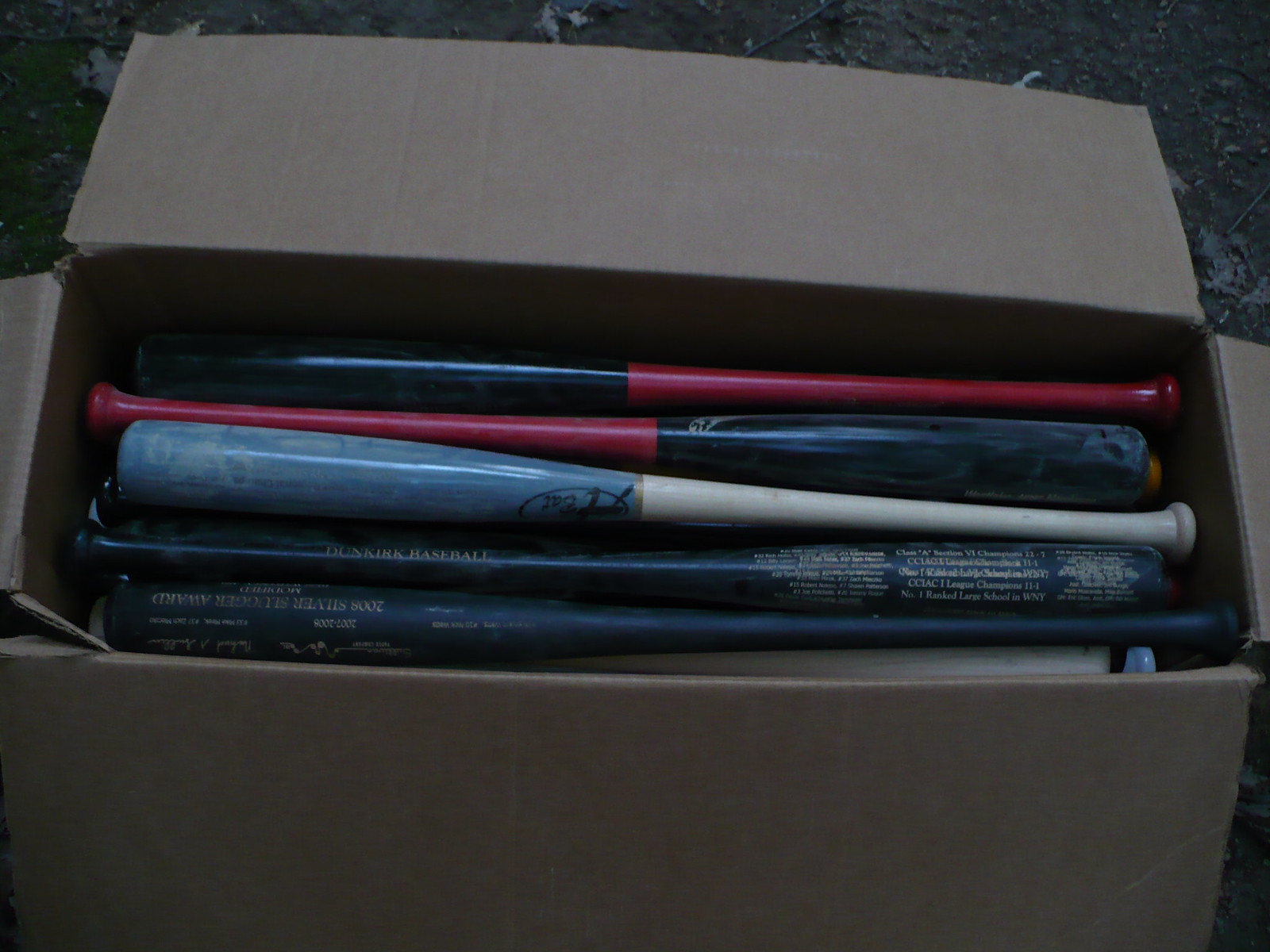The image depicts a long rectangular, open cardboard box filled with an assortment of baseball bats. The cardboard flaps are spread out, with one flap lying flat and the other flaps angled to the sides. Inside the box, the baseball bats are randomly stacked rather than aligned in any particular order. The bats are made of wood and exhibit a variety of colors and designs. Some of the bats have red handles with black upper sections, while others feature white handles paired with blue tops. At least one bat has a brown handle with a blue upper section. Additionally, some black bats display gold lettering, including names like "Dunkirk Baseball." The background of the image is mostly obscured, but a bit of dirt and leaves can be seen around the box. The perspective of the photograph is from above, focusing primarily on the contents of the box.